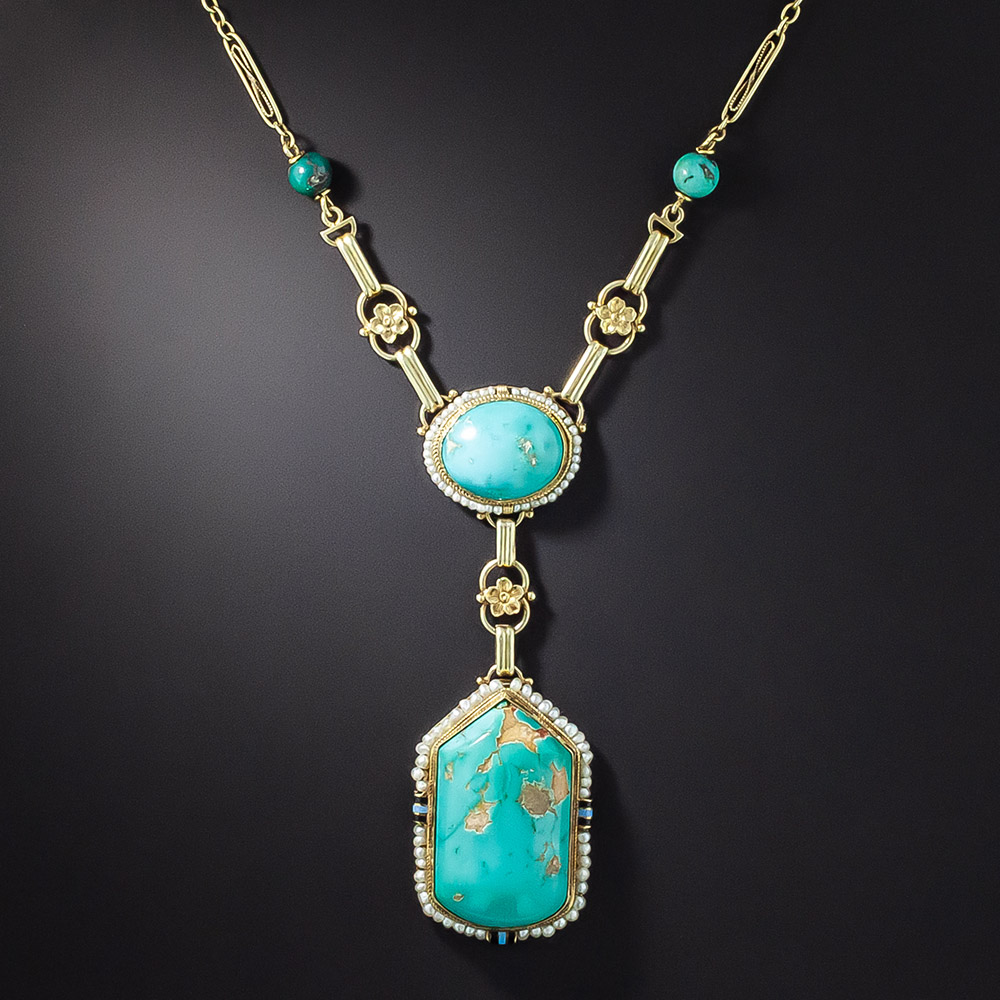This image showcases a well-lit, intricately designed gold necklace against a black background. It features turquoise beads and pearl accents arranged meticulously along the chain. The necklace starts with turquoise beads flanked by sections of gold chain, each connected to flower-link motifs. The centerpiece is a large oval turquoise pendant encircled by delicate white pearls. Attached to this focal point is another pendant, more rectangular in shape with a rounded bottom and a pyramid-shaped top, similarly bordered by white pearls. The gold chain branches off symmetrically to left and right at 45-degree angles, amplifying the elegance of this finely detailed piece.